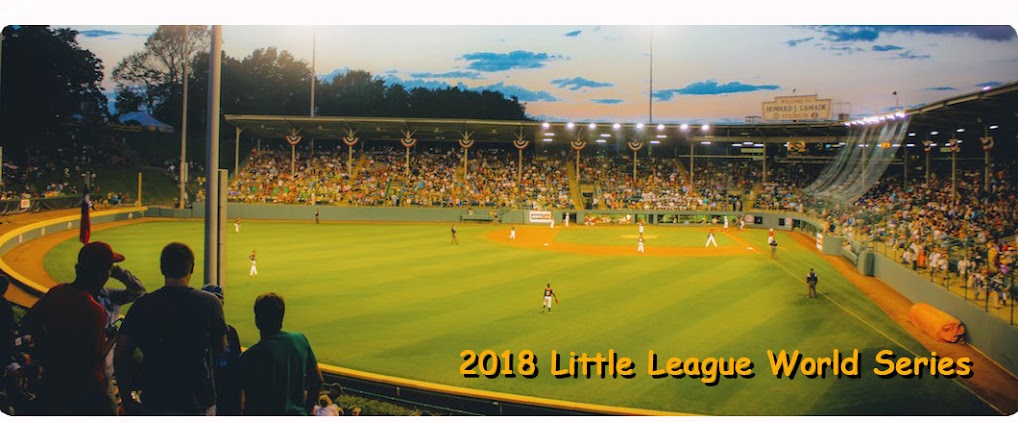The photograph captures the 2018 Little League World Series as noted in the bottom right corner. It was taken from a left-field perspective, giving viewers an expansive view of the field at dusk with the stadium lights illuminating the scene. The sky is dominated by dark clouds, enhancing the contrast with the bright field and dark trees to the left. 

In the foreground, three spectators stand in the bottom left corner, their backs facing the camera. The figure on the left is in red tones with a baseball cap, the middle person is dressed in dark black or navy, and the rightmost individual, slightly lower, wears a green t-shirt. Behind the spectators, other fans fill the covered stands, adding to the bustling atmosphere. 

On the field, boys in uniform are positioned defensively, and the well-maintained field features lush green grass and yellowish sand. In the background, a prominently placed sign reads "Welcome to Howard J. Lamade Stadium," though some text details are partially unreadable. The scene is vibrant yet serene, capturing the spirited ambiance of a Little League game.